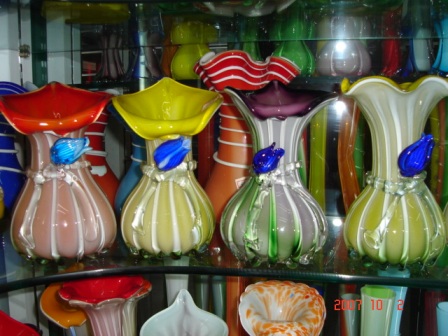In this image, we see a highly detailed display of ornate vases arranged on glass shelves, extending several rows deep into the background. The focal point showcases a series of four distinctive vases, each designed to resemble flowers with intricate veining akin to the petals and undersides of real blossoms. The vase on the far left features a gourd-like shape with a light brown body and vertical white stripes. At the top, an open red flower is blooming, while a smaller blue flower adorns the side. Directly to its right, an almost identical vase has a yellow flower at the top and the same blue flower on the side. The third vase in the series has a silver-gray body with a purple flower on top, also accompanied by a side blue flower. The final vase, which is partially obscured, shares the same design but with a yellow top. Additional ceramic pieces are visible below, including a red-topped piece and a white vase with orange splotches. In the background, various other colored vases can be seen, suggesting a rich and diverse collection. A date, "2007-10-2," is inscribed on one of the ceramic pieces, adding an element of historical context to the display.